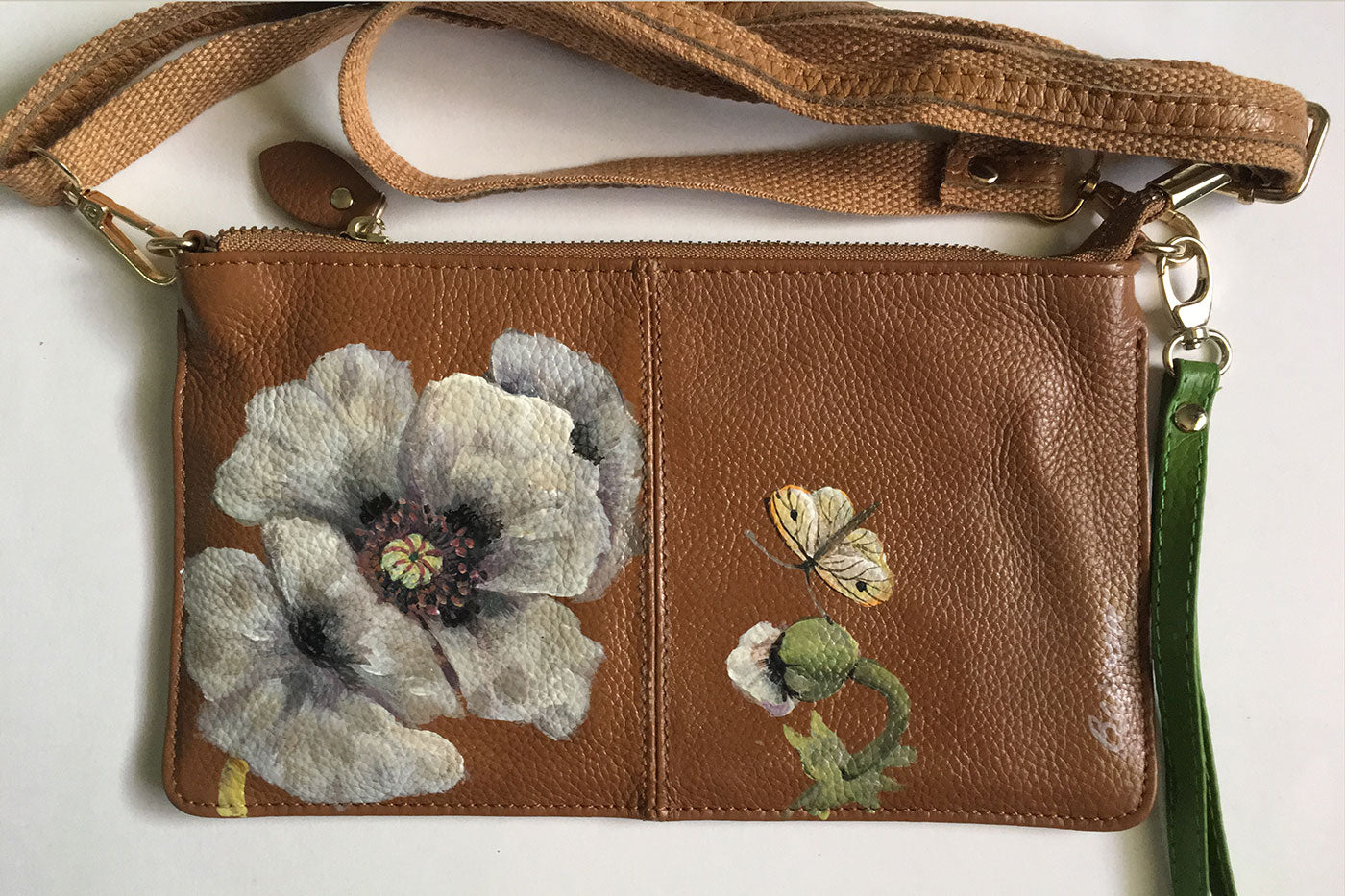This image depicts a close-up of a small, medium-brown purse made of a material that appears to be either leather or cloth. The purse is rectangular in shape with a prominent vertical seam running down its center. On the left side of this seam, there is a detailed depiction of a flower resembling a poppy, which is primarily white and light gray with a touch of yellow and light rose in the center, and encircled by almost black details. Adjacent to the seam on the right side, there is a small green-stemmed flower bud. Hovering above this bud is a small butterfly, characterized by its yellow and black wings. The top part of the purse shows a brown strap that is folded and accordioned together, and there is an additional green strap visible on the right side. The intricate details and careful arrangement of elements on the purse highlight both its aesthetic and functional features.